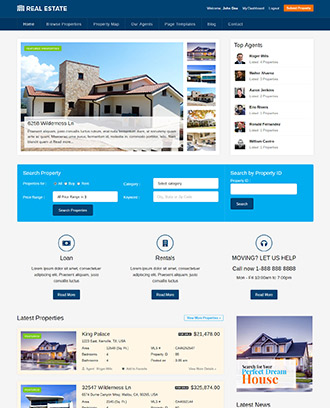This image is a detailed screenshot of a real estate company's website. At the top of the page, there is a blue banner featuring the company's name, which includes the term "Real Estate," along with several clickable menu options for navigation. Beneath this banner, a large, vivid photograph of an impressive stone house with a blue sky backdrop and a substantial chimney is prominently displayed. 

To the right of this main image, there is a vertical column showcasing smaller pictures of other houses. Adjacent to these images, a section titled "Top Agents" features vertically aligned photographs of real estate agents, each accompanied by their names. Below this, a light blue box labeled "Search Property" offers a tool for visitors to search for properties based on criteria such as location and price range.

Further down the page, a gray section provides additional services related to loans, rentals, and moving assistance under the heading "Let Us Help." Lastly, at the bottom of the screenshot, there are several property listings. These include thumbnail images of houses, along with specific details such as location, price, number of bedrooms, and number of bathrooms.